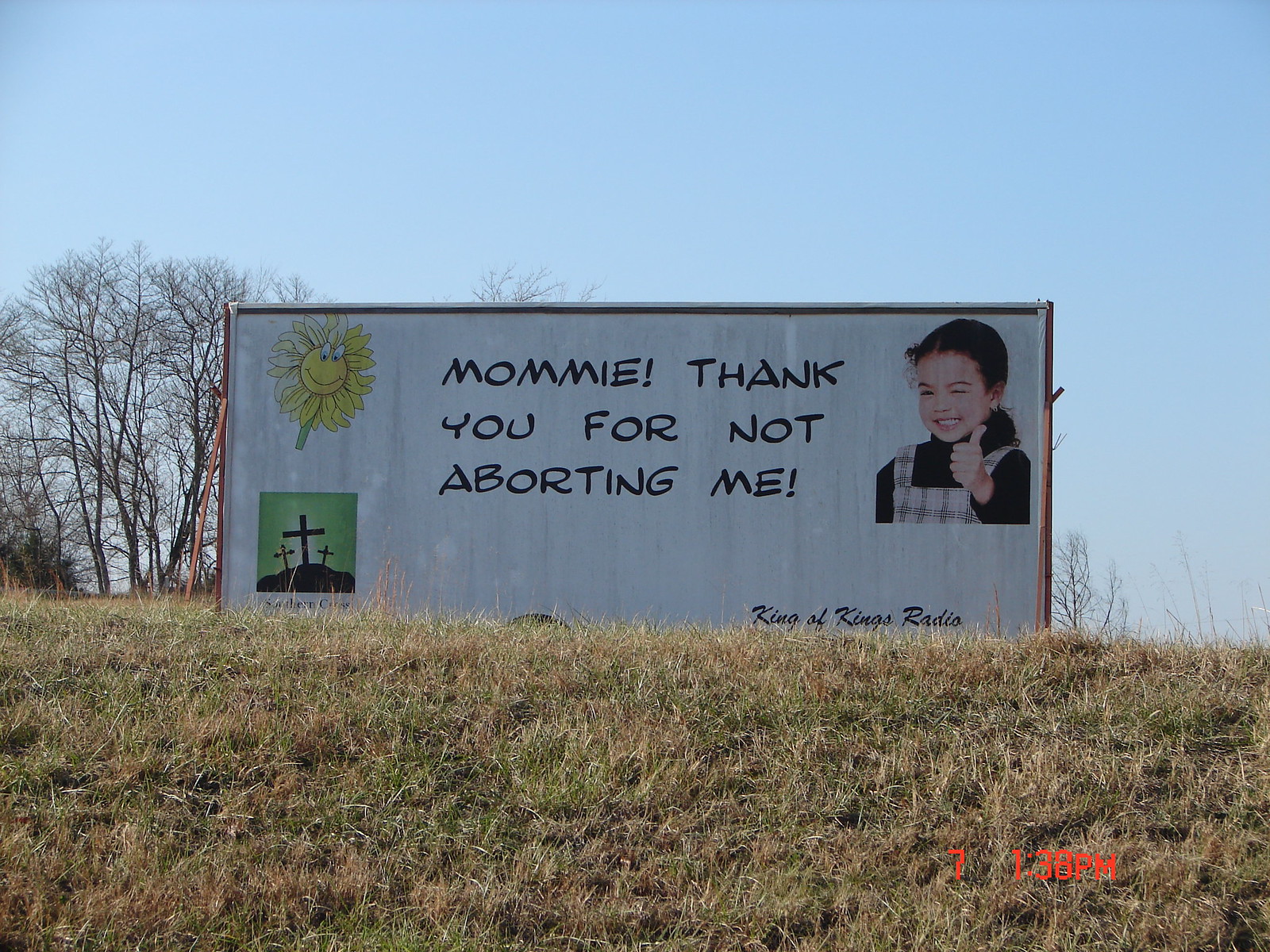This is an image of an outdoor billboard set on a small hill in the middle of a grassy field, with a mix of green and brown worn-out grass. The scene is set during daytime under a clear, bright blue sky. The billboard itself is rectangular and features a white background with a brown wooden frame. 

In the upper left-hand corner, there is a cartoon artwork of a yellow daffodil flower with eyes and a smile. Below that, in the bottom left portion of the sign, a green background depicts three crosses on a hill, reminiscent of gravestones. 

On the top right of the billboard, there is a photo of a young girl with her hair pulled back, her left hand bent at the elbow giving a thumbs up, her left eye winking, and her mouth in a smile. 

The center of the billboard reads, "M.O.M.M.I.E. Thank you for not aborting me!" 

On the bottom right, it says "King of Kings Radio" and also features a timestamp reading "7 1; 3 8 p.m." 

In the background, you can see tall, bare-branched trees with brownish-black trunks. The overall theme of the billboard conveys a religious message.